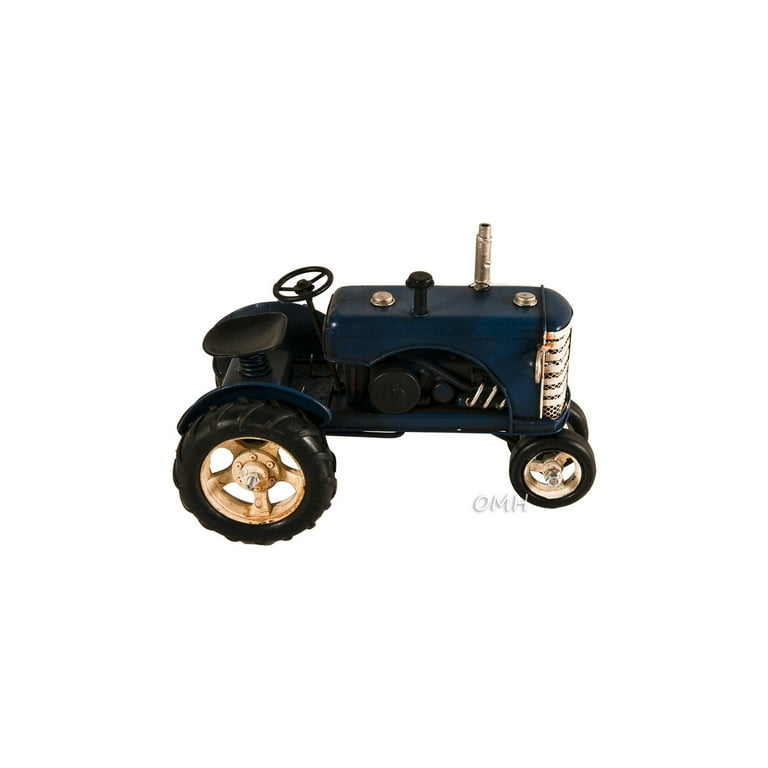The image depicts a miniature toy tractor with a blue body and several black accents, including the seat, steering wheel, motor, and tires. The front tires are smaller than the back ones. The rims have a morphing color that appears to be light, possibly a silvery or goldish hue. Notably, the tractor features a light-colored grill and a smokestack on its side facing away from the viewer. Additionally, some parts, like the diesel cap and bolts, exhibit a mix of rusty white and grayish gold tones. The photo's background is white, and the tractor is oriented towards the right. There is semi-transparent text at the bottom of the image, reading "OMH" in white lettering with a shadow effect, which adds a subtle detail to the overall composition.